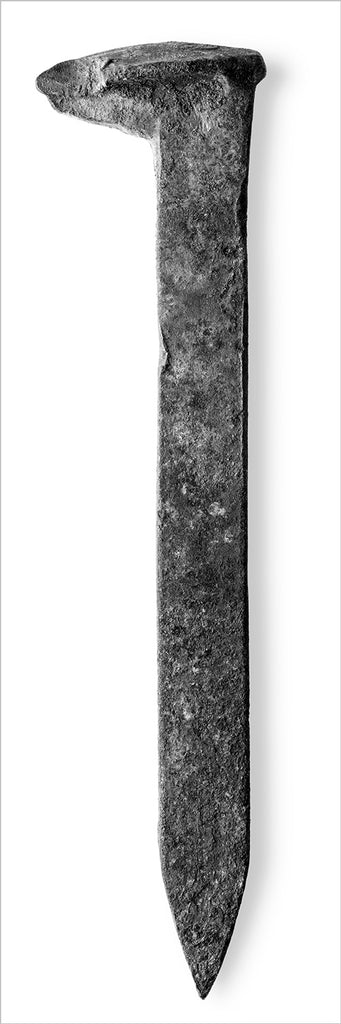The image features a worn, handcrafted railroad spike placed on a white background with a slight shadow beneath it. The spike is predominantly gray, mottled with various shades due to exposure to the elements. It resembles an inverted uppercase "L" with its short, horizontal top extending to the left and a long, vertical shaft descending into a pointed tip. The top left corner of the spike appears to be chipped, possibly from being driven into the ground. The surface of the spike also shows signs of wear, with minor chips and debris scattered along its length, suggesting it has been well-used over time.